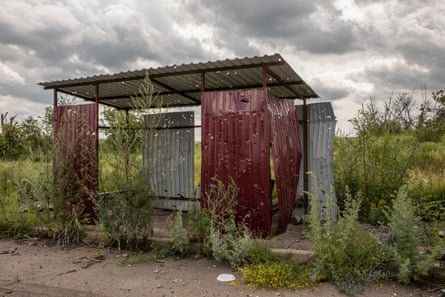The color photograph depicts a neglected outdoor scene under a heavily clouded gray sky. The background reveals an overgrown field filled with tall grass, weeds, and bushes, dotted with debris like rocks and twigs, suggesting long-term neglect. A dilapidated shelter stands prominently in the foreground, constructed from flimsy, corrugated metal plates. The shelter, potentially used as a bus stop, features a mix of gray and burgundy-red metal with a roof designed to offer protection from the elements. The cement road and sidewalk border the shelter, with a visibly discarded paper plate littering the curb, emphasizing the site's abandonment and desolation.